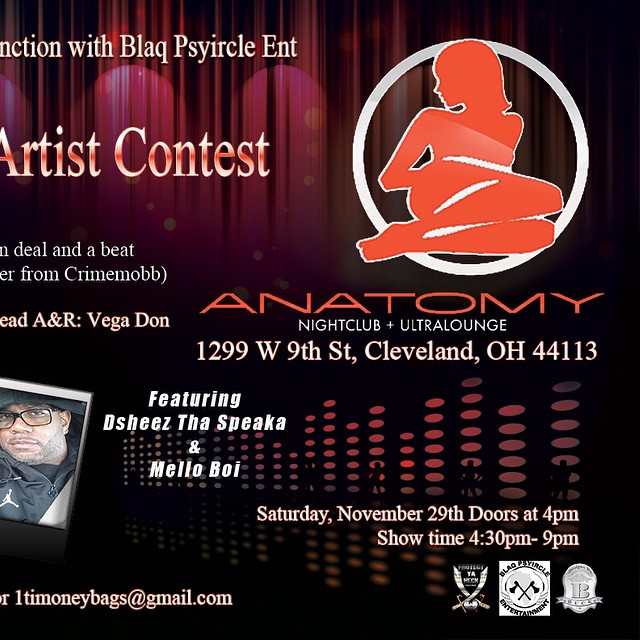This advertisement is for an Artist Contest at the Anatomy Nightclub and Ultra Lounge, located at 1299 West 9th Street, Cleveland, Ohio, 44113. The event takes place on Saturday, November 29th, with doors opening at 4pm and showtime from 4:30pm to 9pm. Featured artists for the night are Deshies, Da Speaka, and Mellow Boi (M-E-L-L-O-B-O-I). The design of the ad includes a mix of black, red, and brown hues, with vertical lines adding texture to the background. A prominent visual element is a white circle at the top right, featuring the red silhouette of a woman sitting with her legs bent and looking over her shoulder. The logo for the lounge, depicted beneath the circle, reads "ANATOMY" in bold red letters, followed by "Nightclub + Ultra Lounge" in white. Additionally, the ad mentions a deal and a beat from Crime Mob and lists Vegadon as the A&R representative. There is also an email address for RSVP and several small, difficult-to-read logos in the bottom right corner, one of which appears to be a symbol with crossed swords, adding to the intricate detailing of the advertisement.